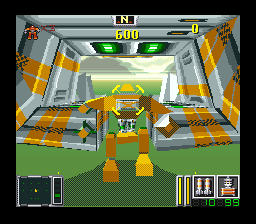This detailed image from a video game features a unique, large character. The character is distinctive with mismatched shoes—one brown and one yellow—and is dressed in brown pants. The character's arms are different colors, adding to its unusual appearance. Its head is disproportionately small compared to its oversized, chalice-shaped torso—narrower at the bottom and wider at the top.

The backdrop of the scene is a transparent, gray space shuttle-like vehicle, adorned with vibrant orange stripes. The transparency of the vehicle allows the ground beneath to be visible, enhancing the realism. In the bottom right corner, green numerals '10' and '99' stand out, while the bottom left corner features a scoreboard-like display. Moreover, there's an image of a small person visible within the space shuttle, adding a layer of intricacy to the setting. The letter 'N' and the number '600' appear prominently beneath the tiny figure.